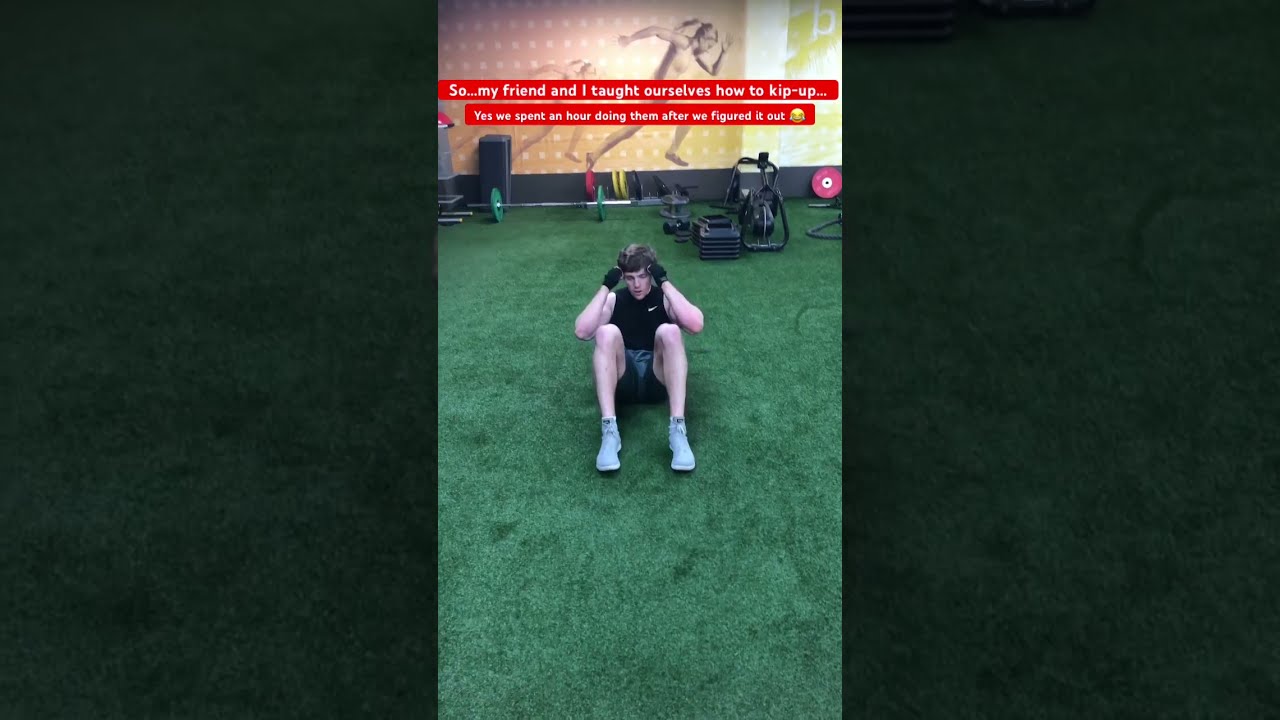In the center of the image, a man with peach skin complexion, brown hair, and wearing a black shirt and gray shoes, is sitting on green turf, appearing to perform crunches. The setting, which seems to be a gym, features an assortment of weightlifting equipment scattered behind him, including black barbells and weight plates in red, yellow, and green hues. In the background, there is a yellow mural depicting a person sprinting across the wall. At the top of the image, a text overlay reads, "So my friend and I taught ourselves to kip up. Yes, we spent an hour doing them after we figured it out." The overall style of the image suggests it is a screenshot from a social media post.